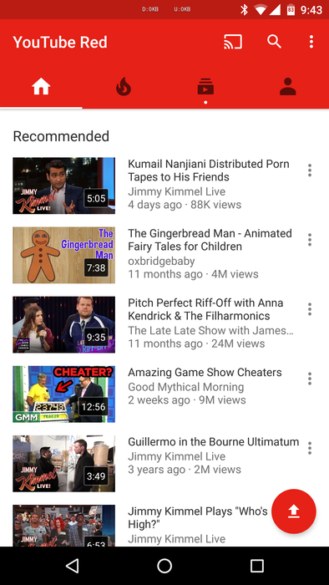This is a detailed screenshot captured on a person’s cell phone, displaying a selection of recommended videos on YouTube Red. Here's a comprehensive overview of the content:

1. The top recommendation features a video titled "Kumail Nanjiani Distributed Porn Tapes to His Friends | Jimmy Kimmel Live." The thumbnail to the left displays Kumail Nanjiani, an Indian-American actor, gesturing animatedly. The video, uploaded four days ago, has accumulated 88,000 views and lasts for five minutes and five seconds. At the bottom left corner of the thumbnail, the Jimmy Kimmel Live logo is visible.

2. The second recommendation is an animated fairy tale for children titled "The Gingerbread Man | Oxbridge Baby." The thumbnail showcases a brightly colored drawing of a gingerbread man smiling widely, with the title "The Gingerbread Man" written in blue letters. This video was uploaded eleven months ago and has garnered four million views. It has a duration of seven minutes and 38 seconds.

3. The third video is "Pitch Perfect Riff-Off with Anna Kendrick and The Filharmonics | The Late Late Show with James Corden." The thumbnail prominently features Anna Kendrick holding a microphone and looking at TV host James Corden. This popular video, uploaded eleven months ago, has received 24 million views and is nine minutes and 35 seconds long.

4. In the fourth position is "Amazing Game Show Cheaters | Good Mythical Morning." The thumbnail shows a game show scene with a contestant standing behind a sign that reads "23743". A game show host looks down at the contestant's winnings while a bold, red arrow labeled "CHEATER" points towards the contestant. The video, with nine million views, was uploaded two weeks ago and runs for 12 minutes and 56 seconds.

5. The fifth video is titled "Guillermo in The Bourne Ultimatum | Jimmy Kimmel Live." The thumbnail depicts Jimmy Kimmel in conversation with his talk show co-host Guillermo, with both men shown in profile. This video, posted three years ago, has two million views and is three minutes and 49 seconds long. The logo for Jimmy Kimmel Live is displayed at the bottom left corner of the thumbnail.

6. The final recommendation is titled "Jimmy Kimmel Plays Who's High? | Jimmy Kimmel Live." The thumbnail features a somewhat blurry image of several people, making it hard to discern specific details. However, the Jimmy Kimmel Live logo is visible at the bottom left corner. This video, which has a duration of six minutes and 53 seconds, does not specify a view count or upload date.

This meticulous snapshot gives a rich overview of a range of diverse and trendy content from the YouTube Red recommendations, complete with timestamps, view counts, and descriptive visuals of each thumbnail.